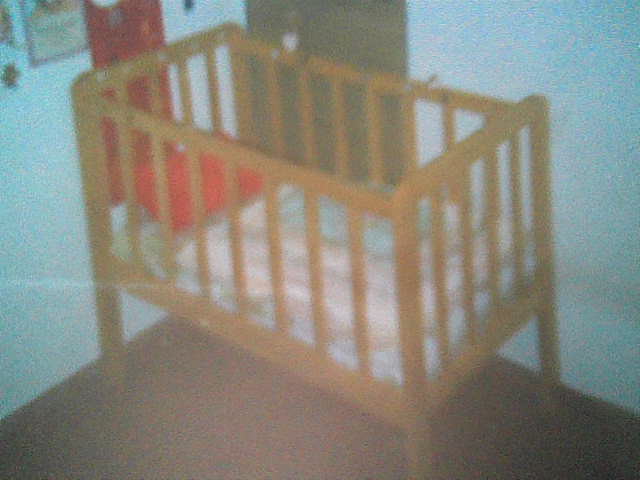A grainy, low-quality photo showcases a simple wooden crib positioned in the corner of a baby room with baby blue walls. The crib features vertical wood bars and contains a red pillow and a light-colored, pinkish-blue blanket. The floor appears to be a brown wooden surface. On the left side of the image, there's a white wall adorned with certificates or pieces of paper, bordered in red. There's also a brownish poster beside the crib. The room is lit with a peculiar lighting effect that blooms in the middle of the picture, adding to the film grain texture apparent throughout the image.